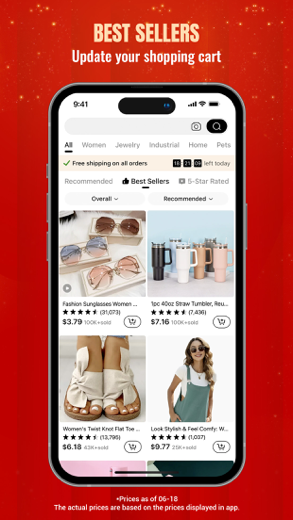In this image, you see a page from an e-commerce website or application displaying various bestsellers. The time on the device shows 9:41, and the iPhone screen depicts icons on the top right, including a full network signal bar, Wi-Fi signal bar, and a fully charged battery indicator. Category options listed on the page include "All," "Women," "Jewelry," "Industrial," "Home," and "Pets." The page offers free shipping on all orders, with a countdown timer indicating 18 hours, 24 minutes, and 4 seconds left for the offer.

Highlighted recommended bestsellers are shown with five-star ratings. The featured products include:
- Fashion sunglasses for women priced at $3.79
- A 40-ounce short tumbler available for $7.16
- Women's twist knot flat-toe shoes costing $6.13
- Stylish and comfy shoes priced at $9.77